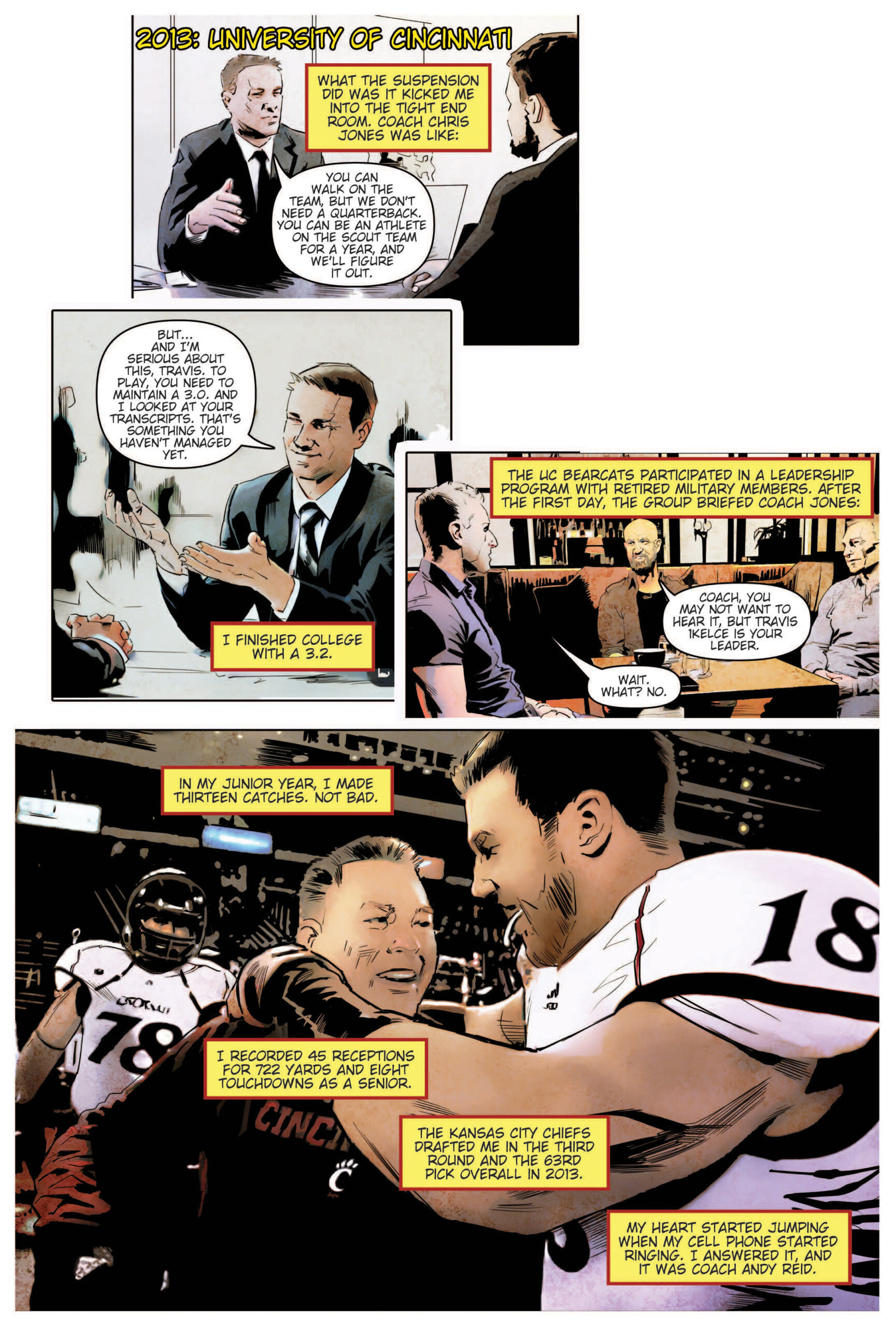This detailed caption is drawn from the key information provided by the three different descriptions:

---

The image is a comic strip, hand-drawn in style and spanning several panels, chronicling the journey of NFL star Travis Kelsey. 

The first panel unfolds in 2013 at the University of Cincinnati, displaying two men in an office setting. One, perhaps a coach or counselor, tells Travis, "What the suspension did was it kicked me into the tight end room. Coach Chris Jones was like, 'You can walk on the team, but we don't need a quarterback. You can be an athlete on the scout team for a year and we'll figure it out.'" Another speech bubble continues, "But I'm serious about this, Travis. To play, you need to maintain a 3.0. I looked at your transcripts. That's something you haven't managed yet." A banner in vibrant red and yellow declares, "I finished college with a 3.2."

Subsequent panels illustrate Travis’s college football progression, detailing his junior year achievement of 13 catches and his senior year accolades of 45 receptions for 722 yards and eight touchdowns. Another key moment captured is the announcement of the Kansas City Chiefs drafting him in the third round, with the 63rd overall pick, in 2013. A climactic panel shows Travis’s excitement as his phone rings and Coach Andy Reid is on the other end, offering him the opportunity to join the Chiefs.

The comic illustrates pivotal moments in Travis Kelsey's career, from overcoming academic hurdles and excelling in college football to becoming a professional athlete in the NFL. Visually, it displays characters in suits against office backdrops, sports action scenes, and celebratory images of Kelsey in a football uniform, marked by the number 18.

---

This narration combines repeated elements, key quotes, and notable visual descriptions, providing a rich, cohesive summary of the comic's content.